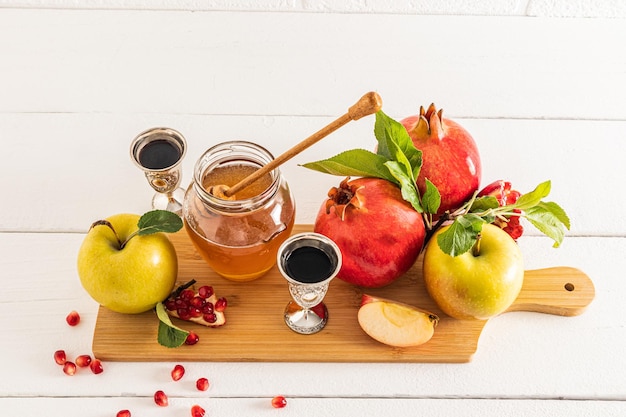This photograph captures a beautifully arranged fruit and honey board set on a rustic, white plank background. The cutting board is laden with a vibrant assortment of fruits, honey, and drinks. On the left side, there's a Yellow Delicious apple and an opened pomegranate with its seeds scattered across the board and table. Central to the display is a large, clear pot filled with golden honey, featuring a wooden honey stick dipped in. Flanking the honey are two elegant small cups, one above and one below, likely holding wine. To the right, there are two whole pomegranates garnished with leaves, a Yellow Delicious apple nearby, and a Red Delicious apple that has been cut open and has started to oxidize. The scene is sprinkled with red berries and further adorned with additional green apples, some with leaves still attached. These elements combine to create a visually appealing and delectable spread, bathed in bright natural light.